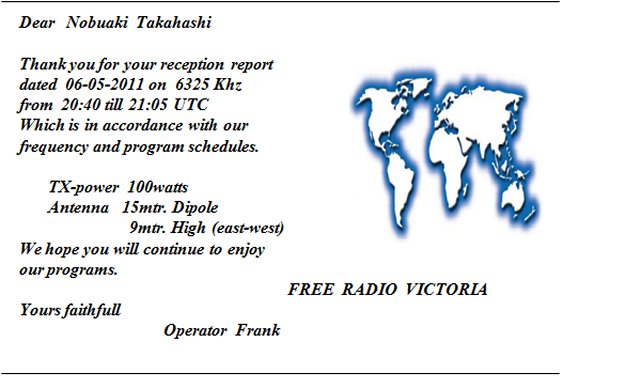The image depicts a formal reception report acknowledgment on a white background, framed at the top and bottom by black horizontal lines. Centered on the right side is a world map outlined in a soft blue hue, highlighting the continents with negative space. The left side contains detailed text which reads: 

"Dear Nobaki Takahashi,

Thank you for your reception report dated 6-5-2011 on 6325 kHz from 2040 till 2105 UTC, which is in accordance with our frequency and program schedules. TX power 100 watts, antenna 15-meter dipole, 9 meters high, east-west. We hope you will continue to enjoy our programs.

Yours faithfully,
Operator Frank."

Below the world map, the text "Free Radio Victoria" is inscribed.